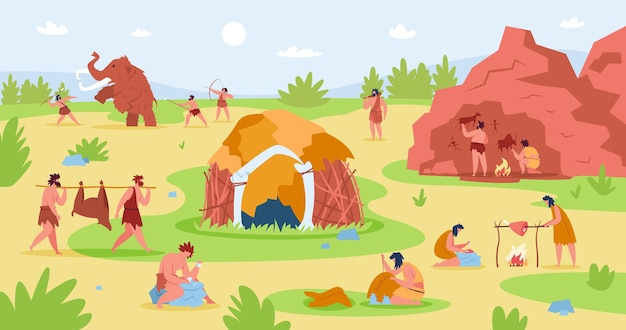The image is a detailed cartoon illustration in portrait mode depicting a prehistoric scene with various activities set in a vibrant landscape. At the top of the image is a light blue sky punctuated with fluffy white clouds. Dominating the middle and bottom sections are hues of yellow, light green, and sandy tones, depicting a rugged environment. 

In the center of the image sits a rounded hut with brown and cream colors, resting on a figure-eight-shaped patch of grass. To the left, two men wearing skirts are seen carrying an upside-down animal by its feet, suspended on a stick between their shoulders. Further left, a dramatic scene unfolds with three people attacking a large mammoth elephant; two wielding spears and one aiming a bow and arrow. 

In the top right corner, amidst pinkish-red rock formations, two individuals are seen painting ancient animal figures inside a cave. Directly below, near a red rock cave, another pair is cooking a side of meat over a fire, enhanced by a verdant green bush and a small blue rock nearby. Additionally, one person is pouring water, adding to the vivid activities displayed.

Towards the bottom center, a woman is engaged in sewing, contributing to the domestic aspect of the scene. The captivating and bustling depiction of early human life is rounded off with a detailed environment of caves, tents, and active inhabitants, presenting a lively glimpse into prehistoric daily activities.